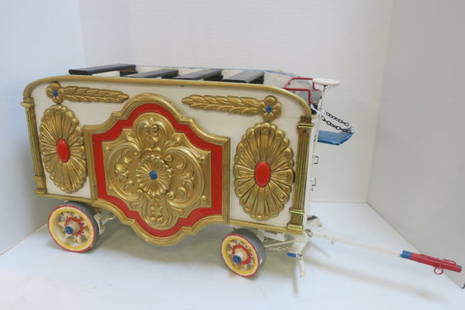This image depicts a detailed model of an old-time horse-drawn wagon, intricately designed and elaborately decorated. The wagon, seated within a small white box-like display without windows, is primarily white with elaborate gold accents and red highlights. The sides are adorned with large, intricate, gold-embroidered panels and crests featuring red gems at both the top corners and the center of the side panels. The cart has yellow wheels with red outlining and blue dots, with the rear wheels being slightly larger than those at the front.

At the front of the wagon, a connecting bar extends outward, ending in a blue tip with a bright red end, likely intended for hitching to horses. The top of the wagon is equipped with black seating arrangements, featuring several rows of benches with low rails, and a folded-down footrest. The wagon's ornate design includes gold pillars on the corners and detailed floral patterns, adding to its decorative appeal. A prominent chain hangs at the front, supporting a blue ornament. This highly decorated model cart, likely used for display purposes, showcases an array of intricate details and craftsmanship reminiscent of historic horse-drawn carriages.